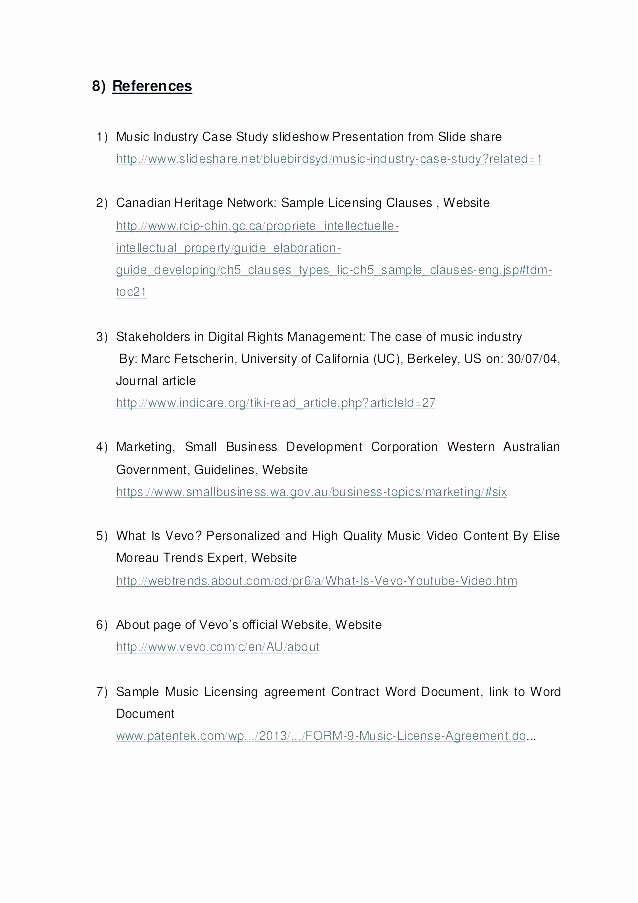The image predominantly features a white background with black and gray text. In the top left corner, the heading "8 References" is prominently displayed and underlined. Below this heading, a numbered list of references is provided along with corresponding gray links. The details of the references are as follows:

1. **Music Industry Case Study Slideshow Presentation from SlideShare**
   - A gray hyperlink follows this description.

2. **Canadian Heritage Network Sample Licensing Clauses Website**
   - Another gray hyperlink is provided beneath this reference.

3. **Stakeholders in Digital Rights Management: The Case of the Music Industry by Mark Fettershorn, University of California, UC Berkeley, US on 3704 Journal Article**
   - A gray link is shown below this entry as well.

4. **Marketing Small Business Development Cooperation Corporation, Western Australian Government Guidelines Website**
   - This reference is also followed by a gray hyperlink.

5. **What is VEVO: Personalized and High-Quality Music Video Content by Elise Moreau, Trends Expert Website**
   - Below this description, a gray hyperlink is provided.

6. **About Page of VEVO's Official Website**
   - Another gray link is listed under this reference.

7. **Sample Music Licensing Agreement Contract, Word Document**
   - A link to the Word document is provided, indicated by a subsequent gray hyperlink.

The image serves as a neatly organized list of references related to the music industry and associated subjects, complete with clickable links for further exploration.